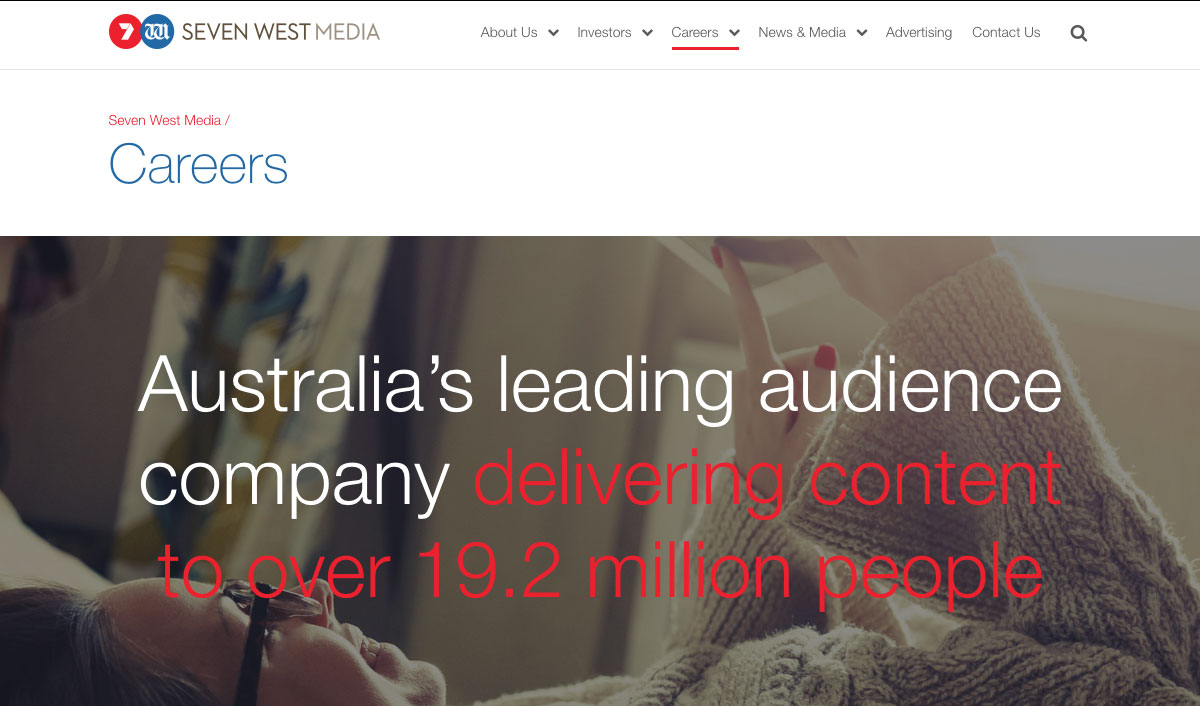This is a website screenshot of Seven West Media. In the upper left corner, the name "Seven West Media" is prominently displayed in capital letters in a gray font. Adjacent to the text is a small pink circle with a white number seven inside it. Next to the pink circle, there is a blue circle featuring white text, which appears to spell out "West."

Moving to the right, the website's navigation menu includes the following options in gray letters with small gray downward arrows: "About Us," "Investors," "Careers," "News and Media," "Advertising," and "Contact Us." There is also a gray search bar. Notably, the word "Careers" is underlined in pink, drawing attention to this section.

On the left side of the page, the text "Seven West Media" is highlighted in pink, with "Careers" written in large blue letters directly beneath it. Below this heading, an image is displayed, featuring a woman lying on her back and holding what appears to be a cell phone. She is wearing glasses and a beige and brown sweater, set against a beige background.

Superimposed on the image are the words "Australia's leading audience company delivering content to over 19.2 million people." The phrase "Australia's leading audience company" is in white letters, while "delivering content to over 19.2 million people" is in red, spanning the width of the image. Below the picture, the background returns to white.